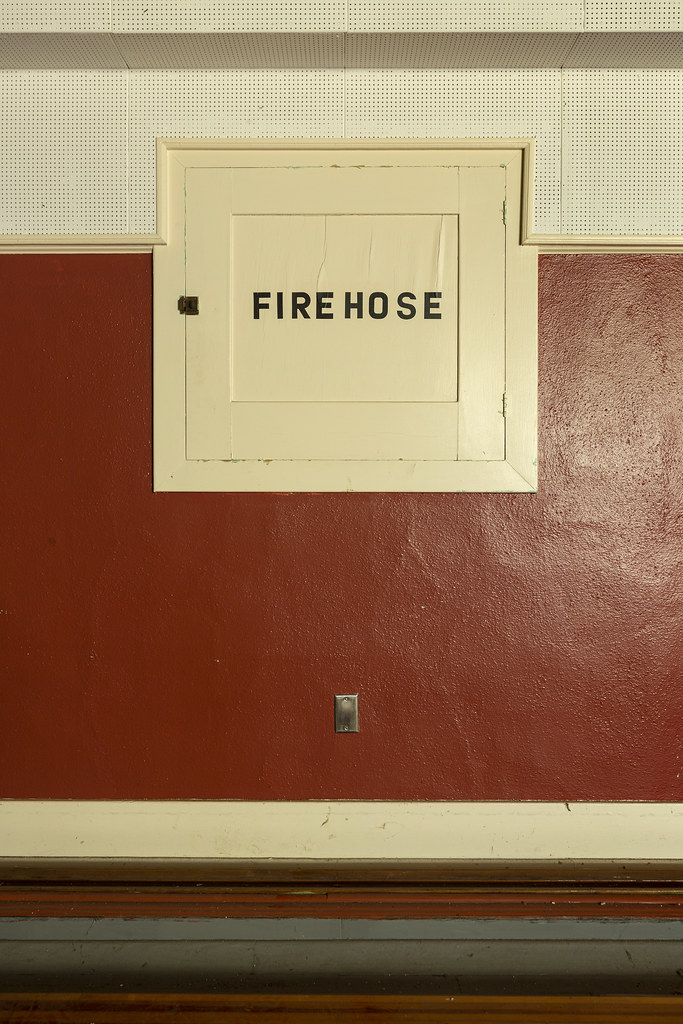This detailed colored photograph, taken indoors, captures a fire hose door mounted on a wall with distinct sections of color and texture. The upper part of the wall has a white textured surface with small squares, transitioning below into a bold brick red color. Below the red section, there is a narrow white strip followed by a wooden beam, and at the bottom, the wall is gray. Prominently in the center of the image is a light cream-colored square door labeled with the words "FIRE HOSE" in large black block letters. The door features visible hinges on the right-hand side and a latch for opening it, presumably to access the fire hose and the water control knob inside. At the bottom of the red section of the wall, there is a silver electrical outlet, adding to the practical details within the composition.